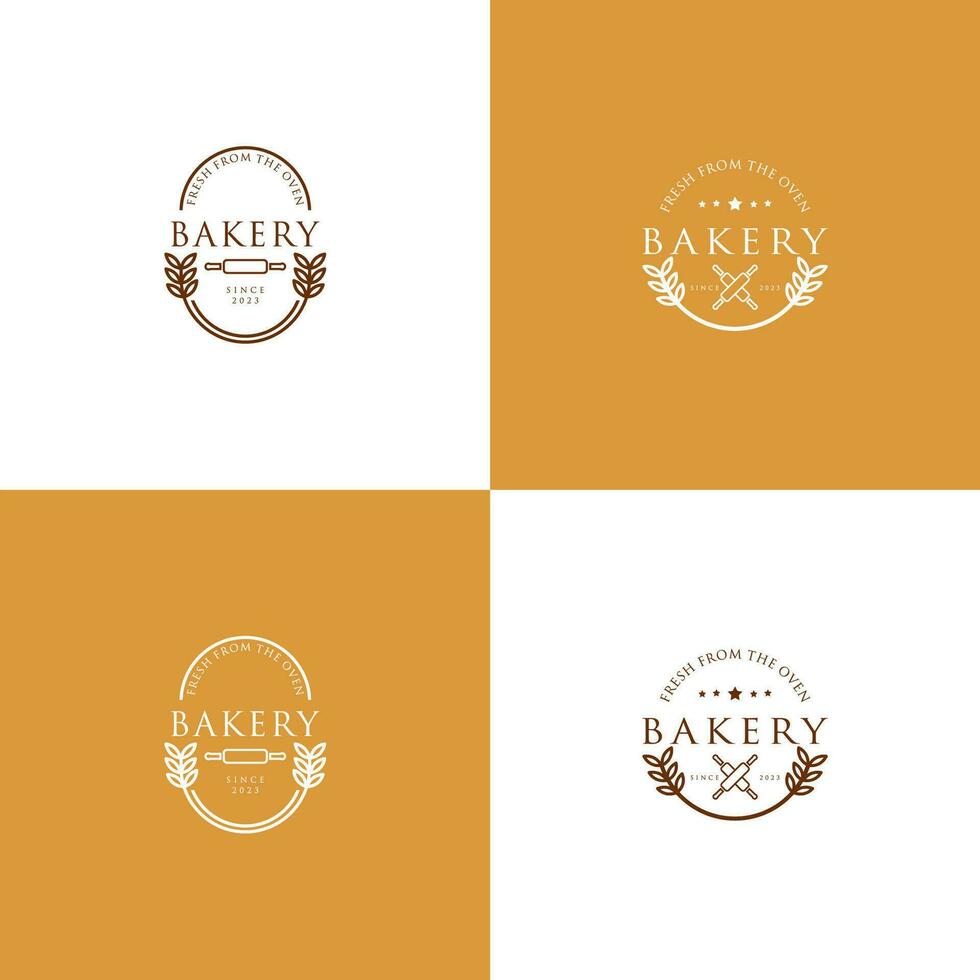The image features multiple versions of a logo for "Fresh from the Oven Bakery." The primary version of the logo is circular, with the text "Fresh from the Oven Bakery" elegantly arranged around the border. At the center, two rolling pins are crossed diagonally, with a delicate flower placed at the intersection, adding a touch of charm and emphasizing the artisanal nature of the bakery. 

In addition to the primary circular logo, there are four alternative versions presented. One alternative retains a similar design but shifts to an oval shape, giving the logo a slightly elongated form. In this version, the central element is simplified to a single rolling pin, still accompanied by the signature flower. The logos are displayed on different background colors, with one set against a white background, enhancing clarity and simplicity, while another is placed on an orange background, evoking warmth and the inviting nature of freshly baked goods.

Each variation maintains the core elements of the brand, showcasing flexibility in design while preserving the essence of the bakery’s identity.